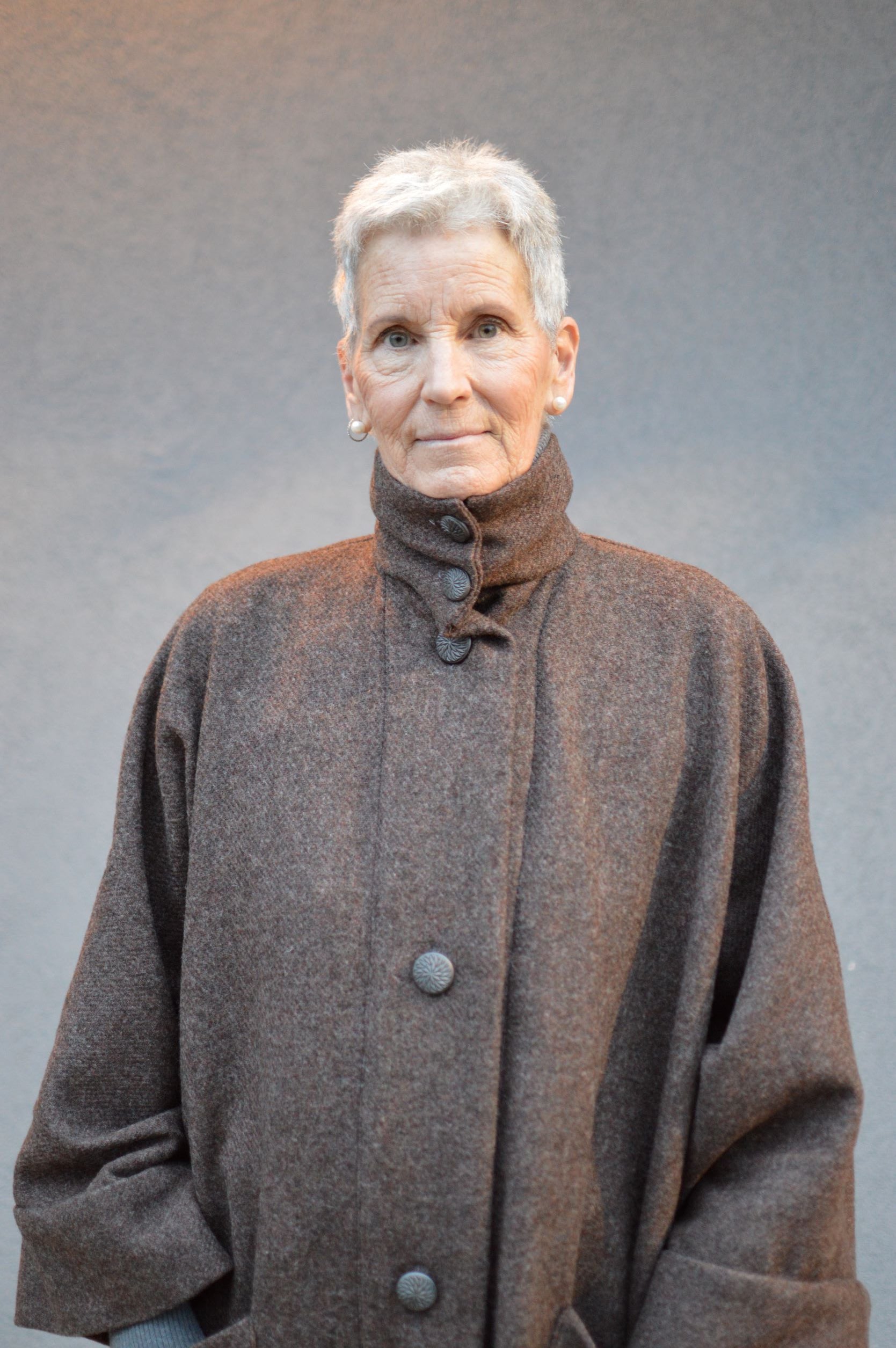This image is a color photograph in portrait orientation, featuring a senior woman modeling an overcoat. The woman has short, grayish-white hair styled very close to the head, giving it an almost masculine appearance. She has a nice complexion and piercing blue eyes. Small pearl earrings adorn her ears, adding a touch of elegance. The overcoat she is wearing is reminiscent of Russian fashion style, made of a thick, light brownish-beige tweed fabric. It features a stand-up turtleneck collar with two buttons that wrap snugly around her neck. Below the collar, three round, fabric-covered buttons run down the middle of the coat, positioned at her collarbone, mid-chest, and probably near her belly button. The coat extends to the middle of her hips and has puffy sleeves that are bell-shaped above the wrists. The backdrop is a gray gradient, complementing the overall tone of the image. The woman appears to be gazing slightly upwards with a half smile on her face, showcasing a subtle but engaging expression. The style of the photograph is representational realism, capturing the textures and details of the fashion item in a clear, focused manner typical of product photography and fashion shoots.